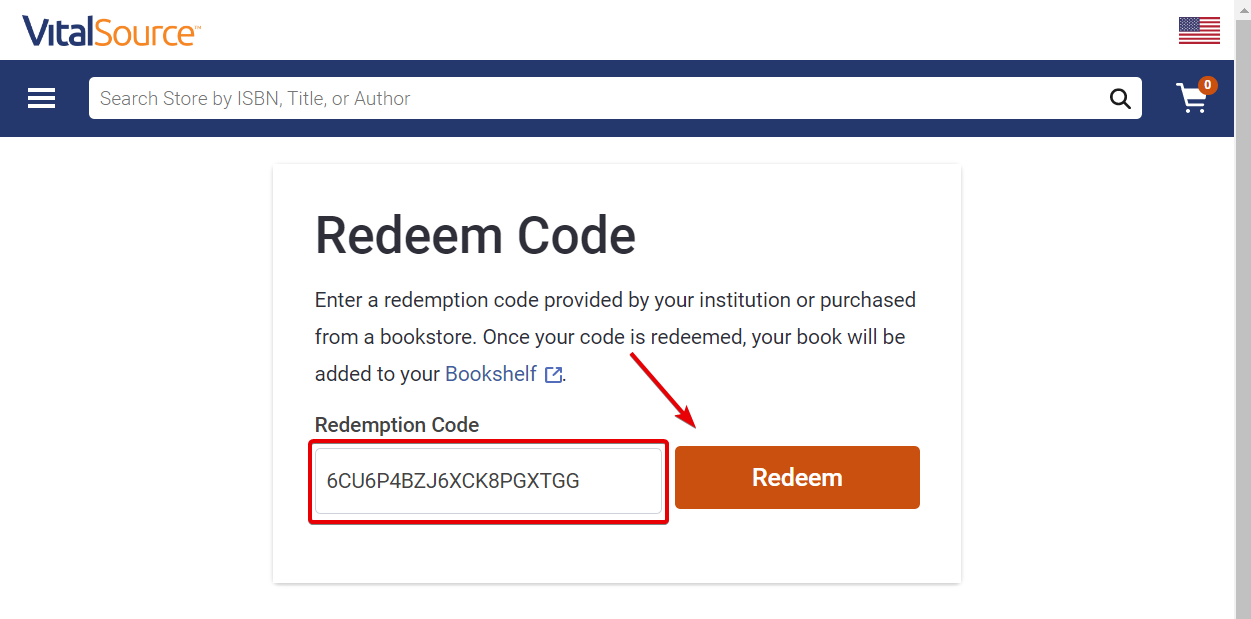The image is a screenshot of a website, specifically from the "VitalSource" page, as indicated by the logo positioned in the upper left corner. The word "Vital" is capitalized in blue text, and "Source" is capitalized in a yellowish-orange text adjacent to it. In the upper right corner, an icon of the American flag is displayed alongside a partial description of its field.

Below the logo and flag icon, there's a search bar with a blue background. It contains a menu icon symbolized by three horizontal lines. Beside this, there is a white text box that reads, "Search store by ISBN, title, or author." At the far right of this box is a magnifying glass icon. Additionally, there is a shopping cart icon with a small red circle and a zero in its center, indicating there are no items in the cart.

Directly below this search area is a prominent text box with bold black text stating "Redeem code." Smaller text beneath provides instructions: "Enter a redemption code provided by your institution or purchased from a bookstore. Once your code is redeemed, your book will be added to your bookshelf." The word "bookshelf" is highlighted in blue with a small square icon featuring an arrow pointing to the upper right corner. 

Below this instructional text, a field labeled "Redemption code" is present, showing a code highlighted in red: "6CU6P4BZJ6X6K8PGXTGG." To the right of this code field is a redeem button with a red background and white text, further emphasized by an arrow pointing towards it.